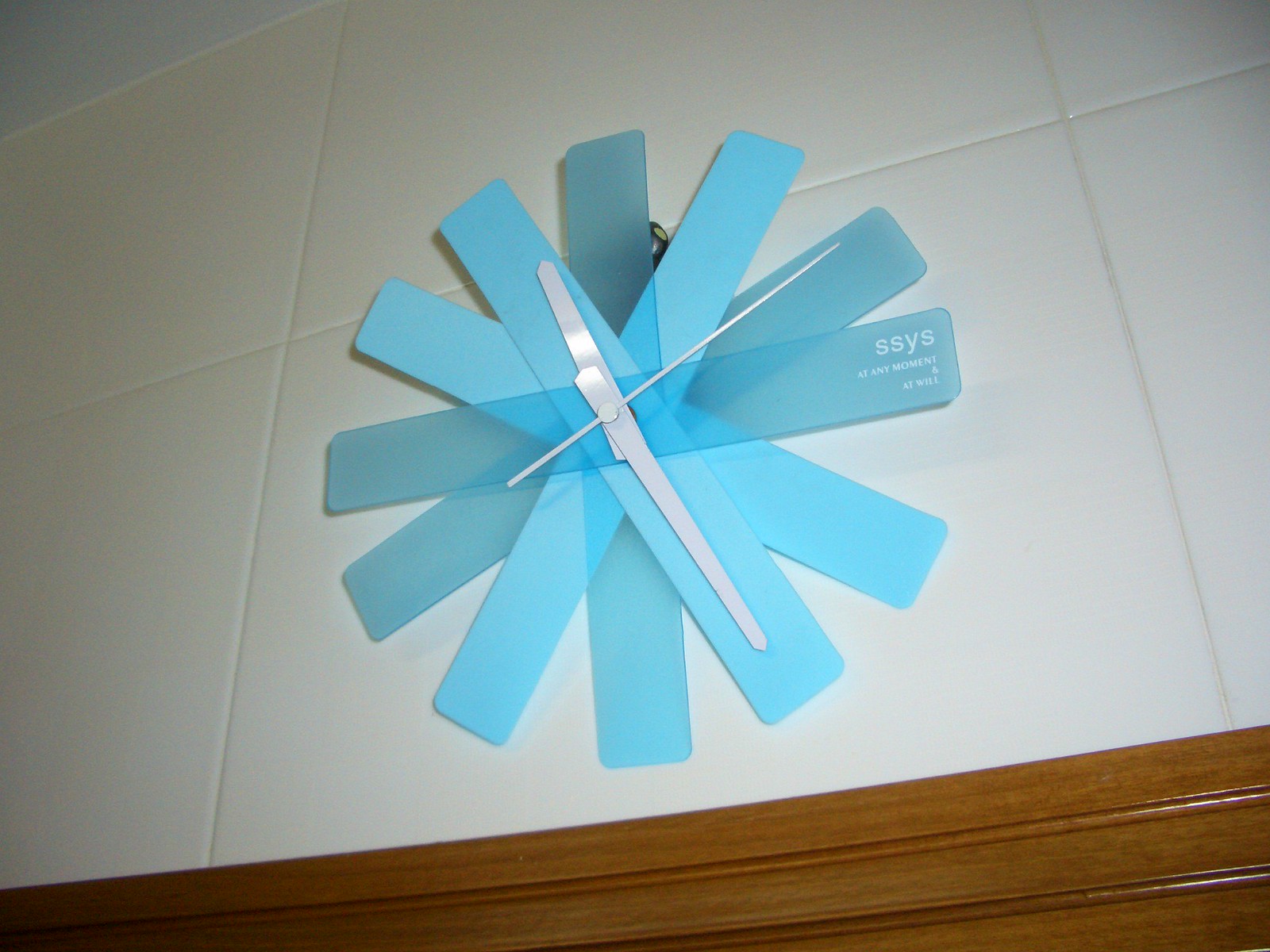This image showcases a unique and artistic wall clock crafted from strips of blue plastic. These strips are arranged in an overlapping manner to form a perfect circle, with each strip representing an hour on the clock. The strips, each about an inch wide, span from one hour to the corresponding opposite hour— for example, a strip extends from 12 o'clock to 6 o'clock, another from 1 o'clock to 7 o'clock, and so forth. This creates a visually intriguing pattern as they radiate around the clock face.

The clock's hands are distinguished by their delicate design; two fine, white strips indicate the hour and minute, while an even finer strip serves as the second hand. Adding a touch of subtle detail, one of the blue plastic strips is inscribed with the letters "SS" and text beneath them, enhancing the clock's distinctive character.

The clock is mounted on a wall adorned with ceramic tiles, which provide a smooth and clean backdrop. Below the tiled wall, a wooden plinth adds a contrasting element of warmth and texture to the scene, grounding the clock within a composed and stylish setting.